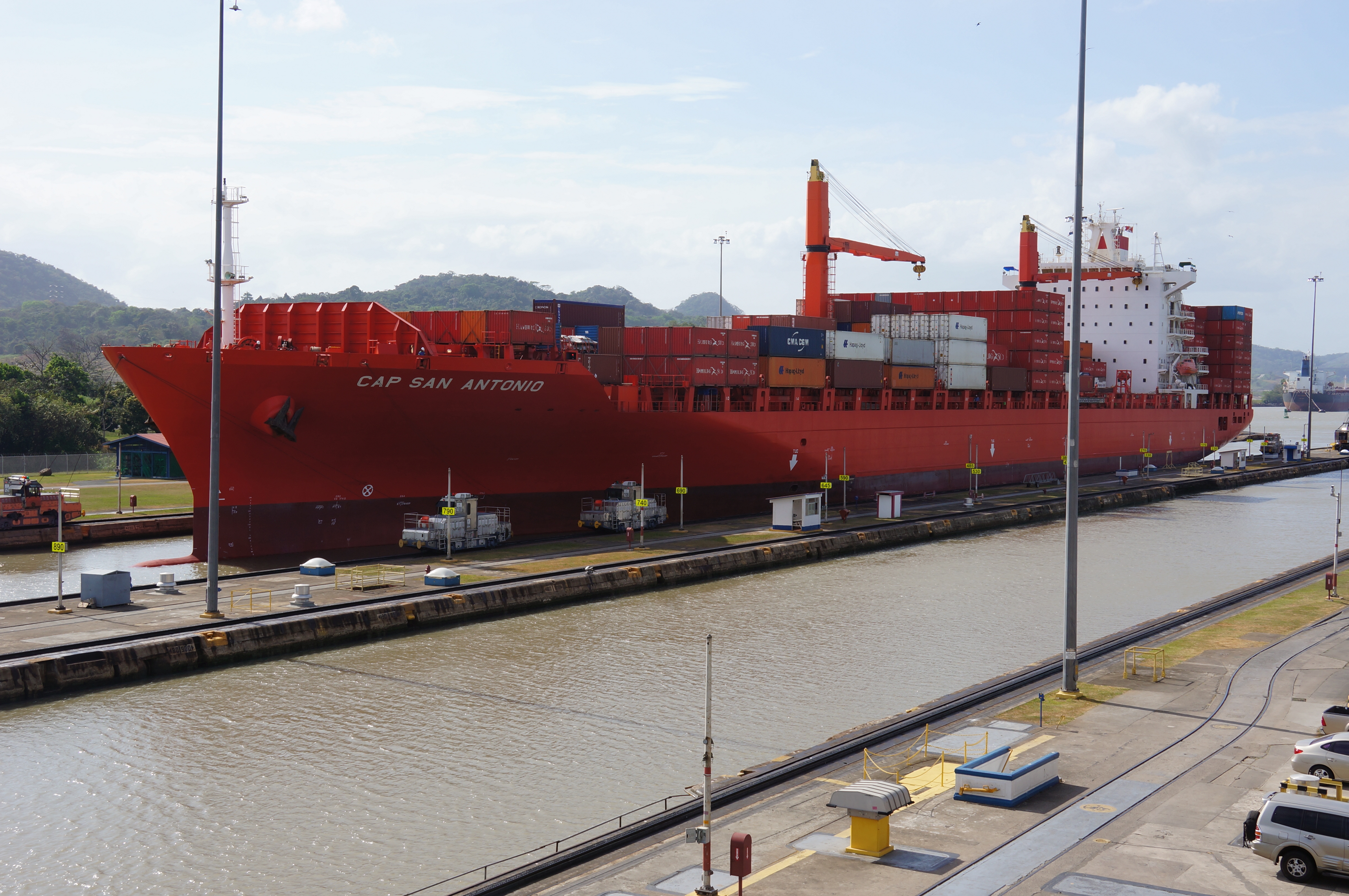The image showcases an outdoor scene beneath a light blue sky dotted with white, puffy clouds. In the background, a scenic mountain range or hills stretches across the horizon. Dominating the foreground is a red container ship named "Cap San Antonio," which exhibits a bright red hue above the waterline and a darker red below. The vessel is stacked with numerous cargo containers in various colors, primarily red, with some white, orange, and blue ones mixed in.

The ship is docked at a canal-like dock, adjacent to a concrete walkway. Alongside the dock, there are red container-picking arms and a white tower with windows where the ship's personnel operate. In the space between the ship and the dock is another body of water, highlighting the dock's multi-waterway nature.

To the right of the image, there is a concrete area with tracks and several parked cars. This area appears to be part of the logistical infrastructure supporting the dock operations. Small cabins are also scattered along the dock, emphasizing the bustling activity in this port setting.